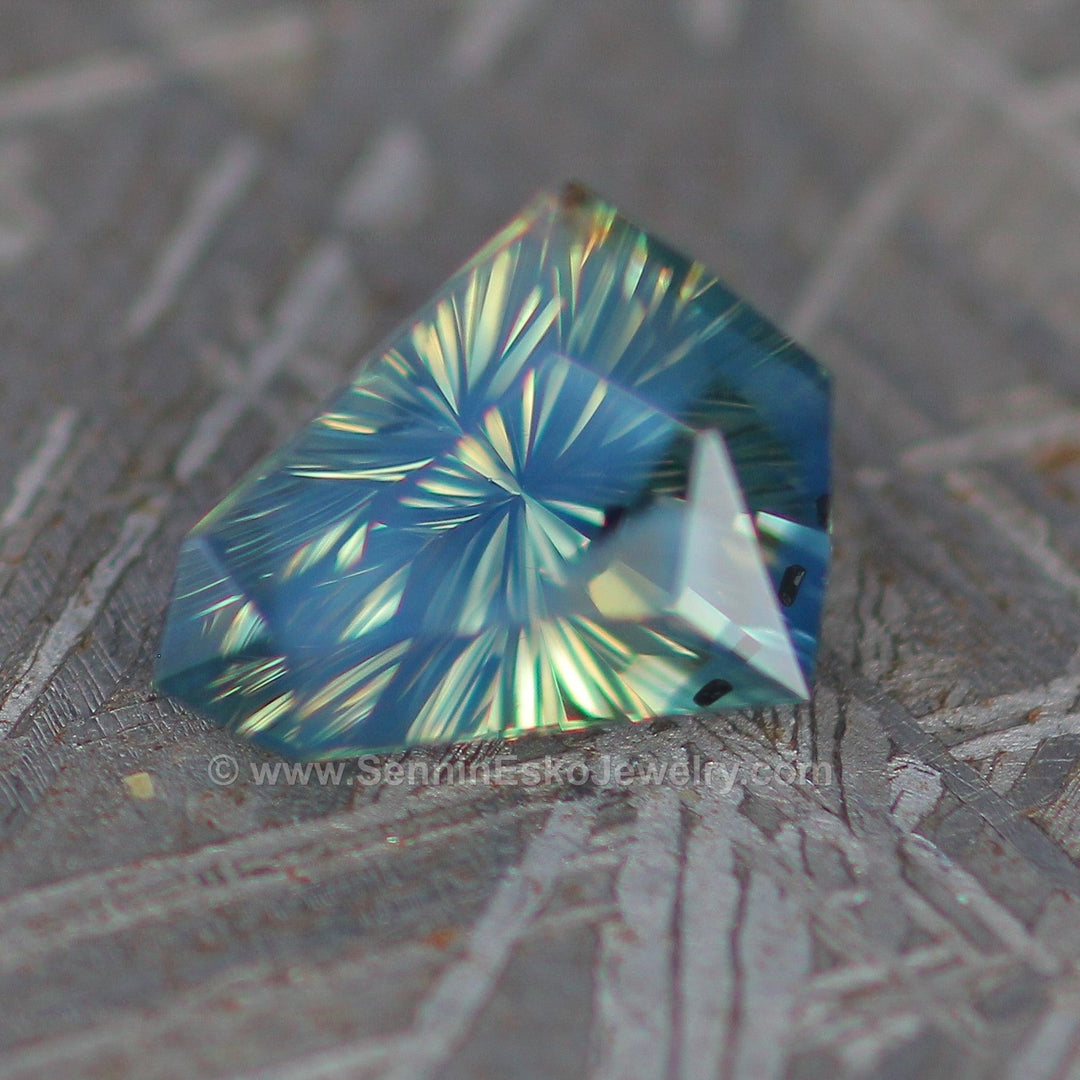The image features a high-end, faceted gemstone that exhibits a striking interplay of colors, primarily yellow with hints of blue and green. The gem, positioned against a gray, unadorned background, reflects light in a way that adds to its multifaceted allure. Surrounding the gemstone are subtle gray markings, enhancing its vibrance and clarity. A watermark across the center of the image reads "www.sennenescojewelry.com," anchoring the visual focus and underscoring its association with an upscale jewelry brand. Though the exact type of gem is ambiguous, it clearly stands out as a luxurious and mesmerizing piece.